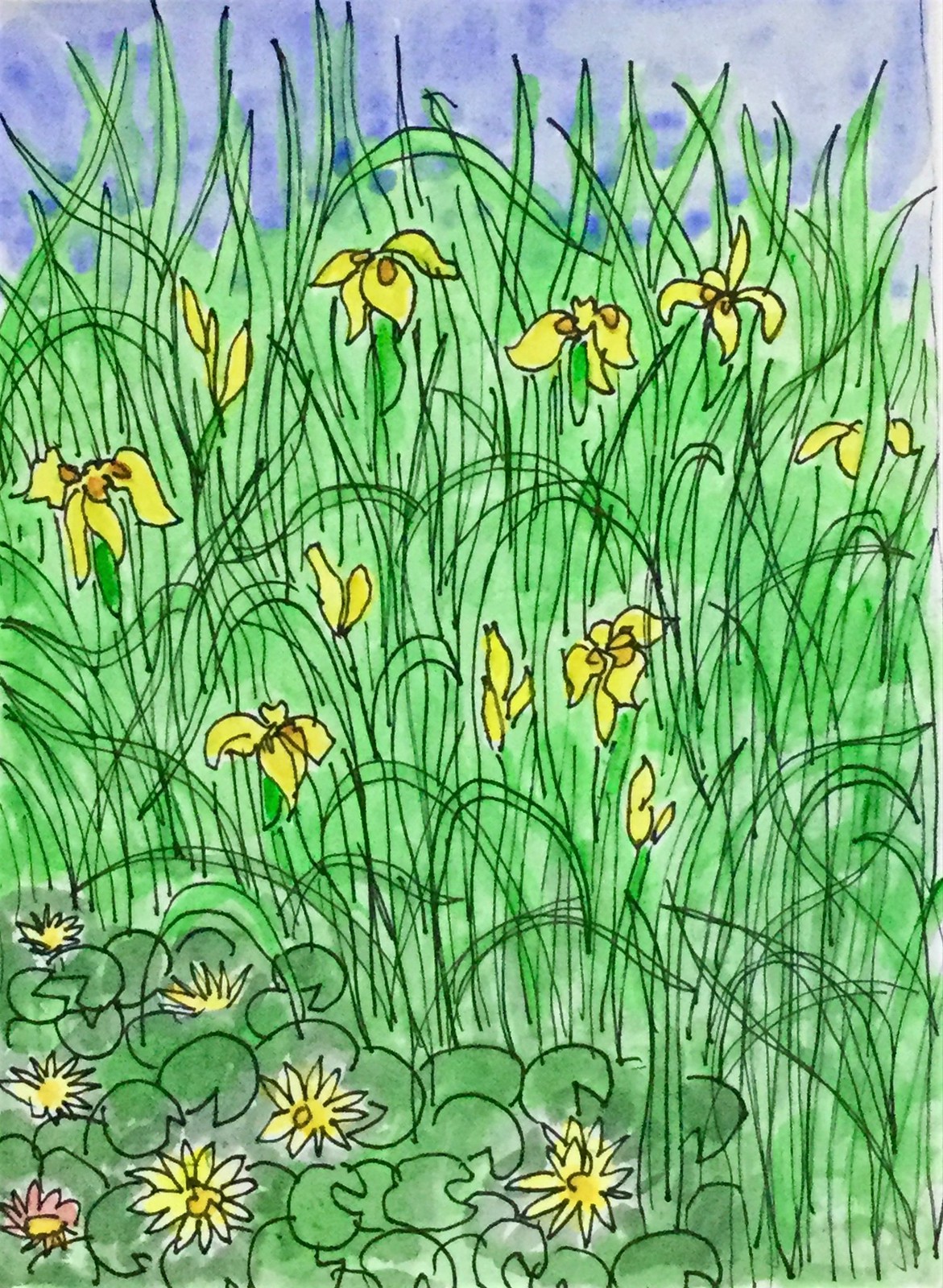This artwork portrays a serene grassy field abundant with vibrant yellow flowers scattered across the landscape. At the bottom, there are lily pad-shaped green leaves interspersed with spiky, yellow-flowered plants and a striking red flower with a yellow center that stands out as an oddball among its yellow counterparts. The midsection features long, wispy grass stalks, some folded over, accompanied by yellow flowers with darker orange centers that resemble irises and droop gracefully. The upper portion showcases a blue sky, varying in tone from darker to lighter, adorned with white clouds, adding to the tranquil ambiance. The entire piece appears to be outlined with black ink and brought to life with delicate watercolor paints, adding depth and subtlety to this detailed and textured scene.